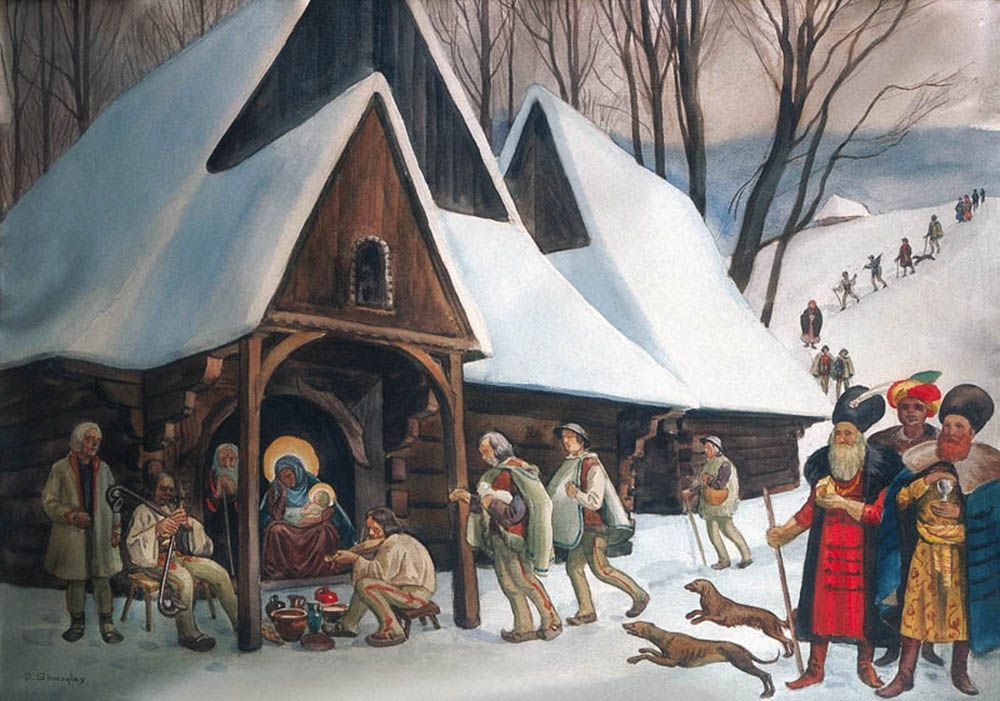A horizontal-rectangular image depicting a detailed and nostalgic manger scene, reminiscent of early 1900s Western European art. The centerpiece is a large, dark wooden stable with peaked roofs blanketed in white snow, situated predominantly on the left to middle portion of the image. Inside the stable, underneath an awning, sits Mary with a halo around her head, tenderly holding the baby Jesus. Outside the stable, various people are gathered, each contributing to the serene atmosphere. In the lower right, three men dressed in colorful clothing, resembling Balkan royalty, present their gifts, symbolizing the three wise men. Two brown dogs rush excitedly towards the manger. On a wooden bench under the awning, an individual plays a musical instrument, surrounded by containers and other seated figures. Behind the stable, a snowy path leads more visitors toward the holy family, all set against a backdrop of snow-covered trees.